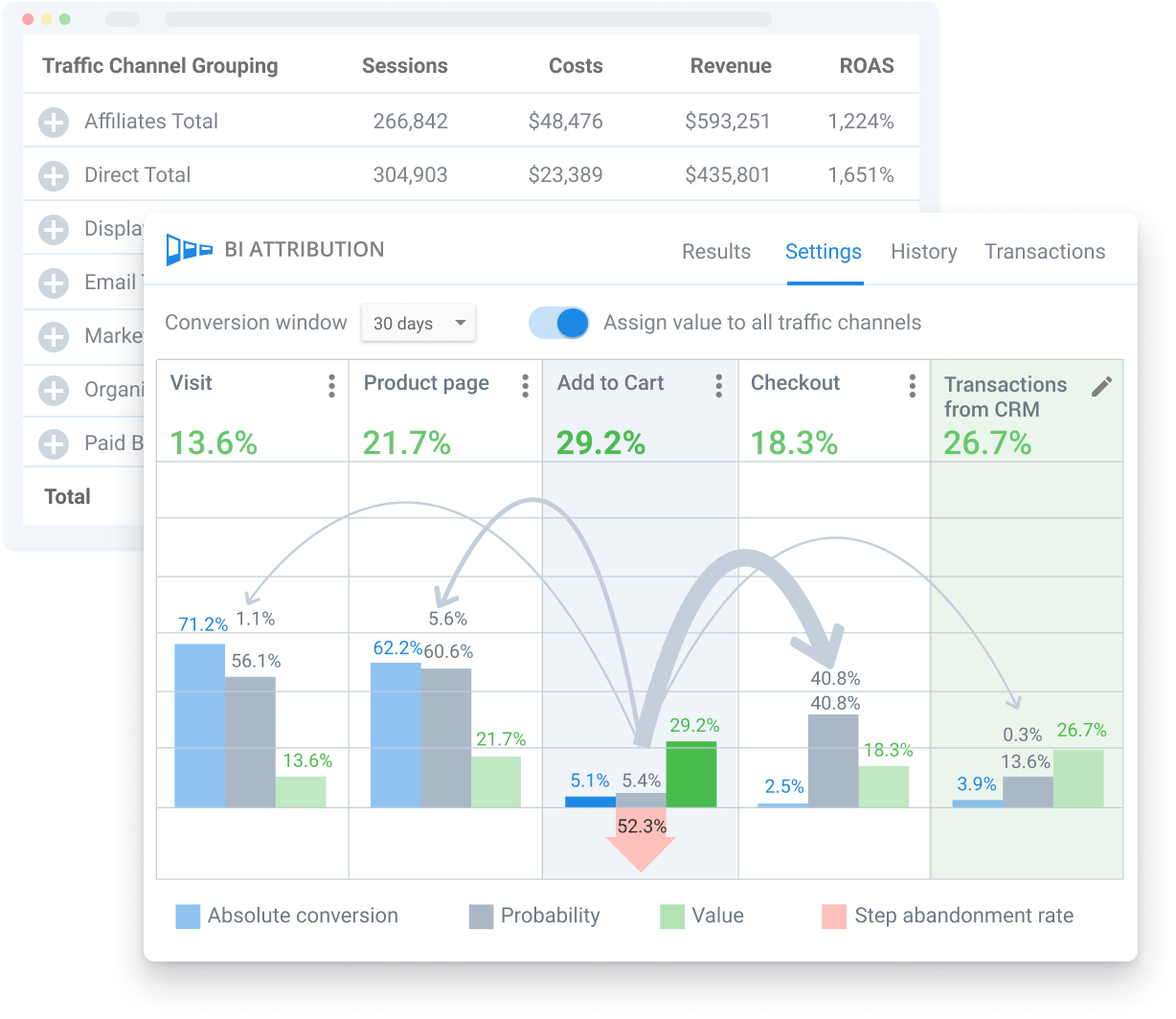The image depicts a detailed interface on a white background. In the upper left corner, there is a prominent blue rectangle with a white inner rectangle. Overlapping this, and covering the bottom right portion and extending slightly more than halfway up, is a large white square.

Within the top white square, an icon is located in the upper left corner. Below it, the text "BI Attribution" is written in gray. To the right, a horizontal menu bar features options labeled "Results," "Settings" (highlighted in blue and underlined), "History," and "Transactions." Beneath this menu, the phrase "Conversion Window" is displayed alongside a drop-down box that currently reads "30 days." Next to this drop-down, there is a blue toggle switch in the "on" position, labeled "Assign value to all traffic channels."

Further down, the interface presents five vertical rectangles with respective labels: "Visit," "Product Page," "Add to Cart," "Checkout," and "Transactions from CRM." Each rectangle is accompanied by percentages in green underneath. At the bottom, a graph with arrows connecting the rectangles visually represents data flow.

Enclosed within the white square, there are five columns of data. These columns are titled "Traffic Channel Grouping," "Sessions," "Cost," "Revenue," and "ROAS." The data within these columns is partially obscured and difficult to read due to being cut off.